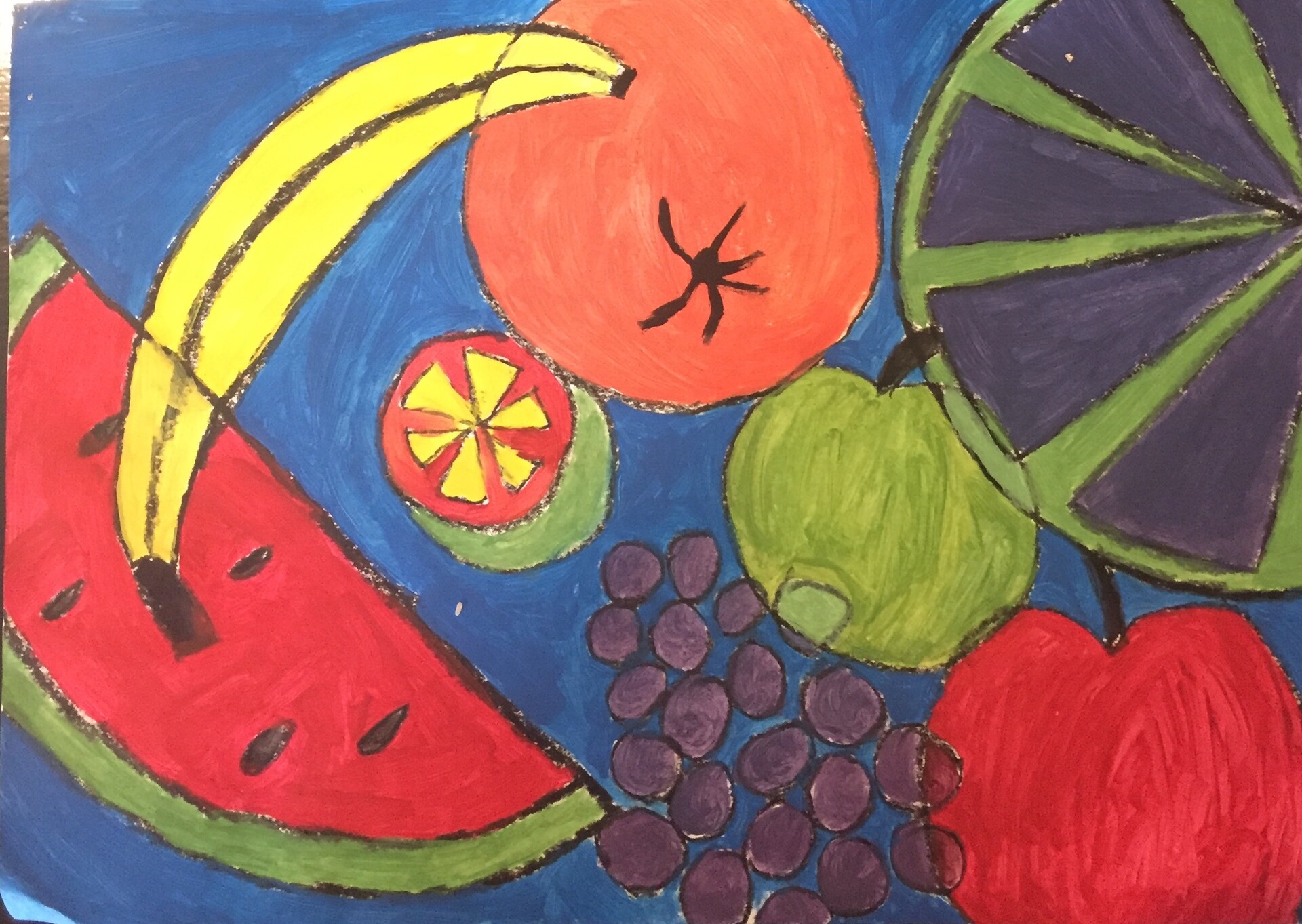This vibrant painting, possibly done in oil or magic marker, features a colorful collage of fruits against a swirling blue background. From left to right, there's a wedge of watermelon with a green rind and tiny black pits, followed by a curved yellow banana with a brown line. An orange sphere with a spider web-like black top lies next to a red fruit with yellow triangles, possibly a tomato or grapefruit slice. To the right, a green apple with a black tip sits beside a cluster of purple grapes, and a larger red apple with a brown stem. Finally, a giant green lime wedge with intricate, dark blue or purple triangles completes the arrangement. The painting's vivid colors and dynamic brushstrokes evoke a Van Gogh-like, relaxing ambiance.